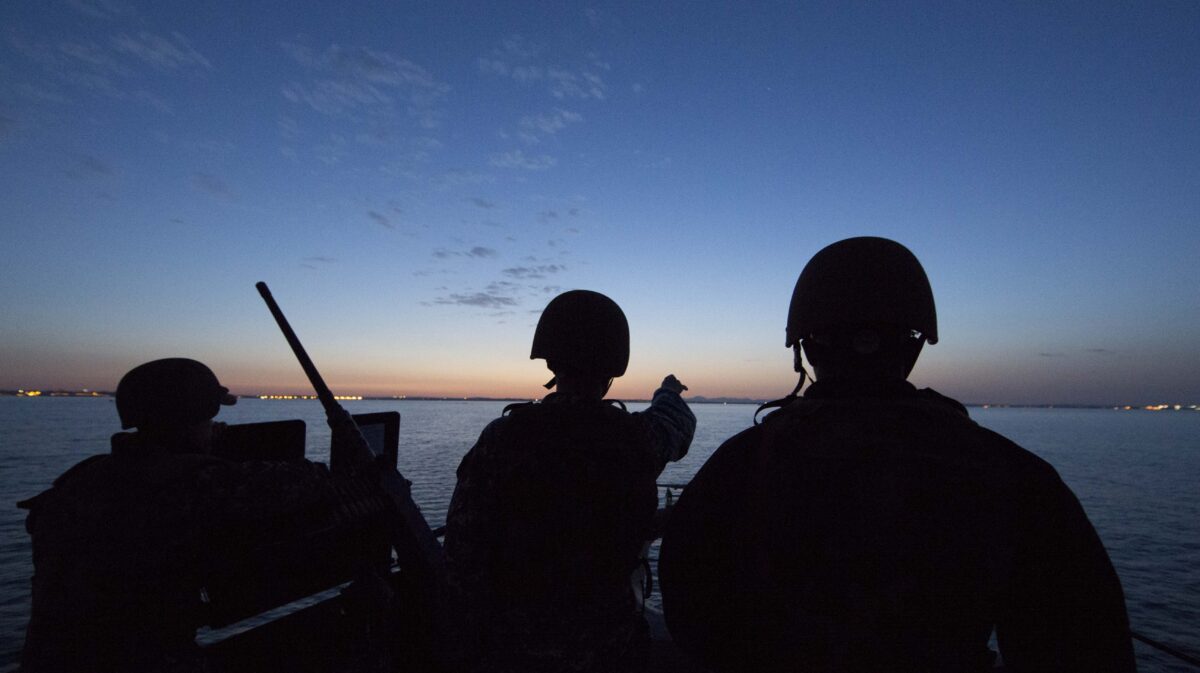In this outdoor photograph taken at dusk, we see the silhouettes of three helmeted soldiers standing on a military boat, their backs facing the camera. They are illuminated only by the fading light of the setting or rising sun, which creates a soft glow in the sky that transitions from a darker blue to a hint of yellow at the horizon. A large gun turret juts out to the left, angled towards the upper left corner of the image. The soldier in the center is gesturing out across the calm, open waters, possibly pointing towards a distant target or their intended direction. The far horizon is dotted with faint, scattered lights, suggesting the presence of a distant township. The scene is bathed in the serene yet somber atmosphere of twilight, with clouds casting gentle shades across the sky. The overall mood is one of vigilant watchfulness, as the men stand still, their figures sharply outlined against the dusky backdrop.